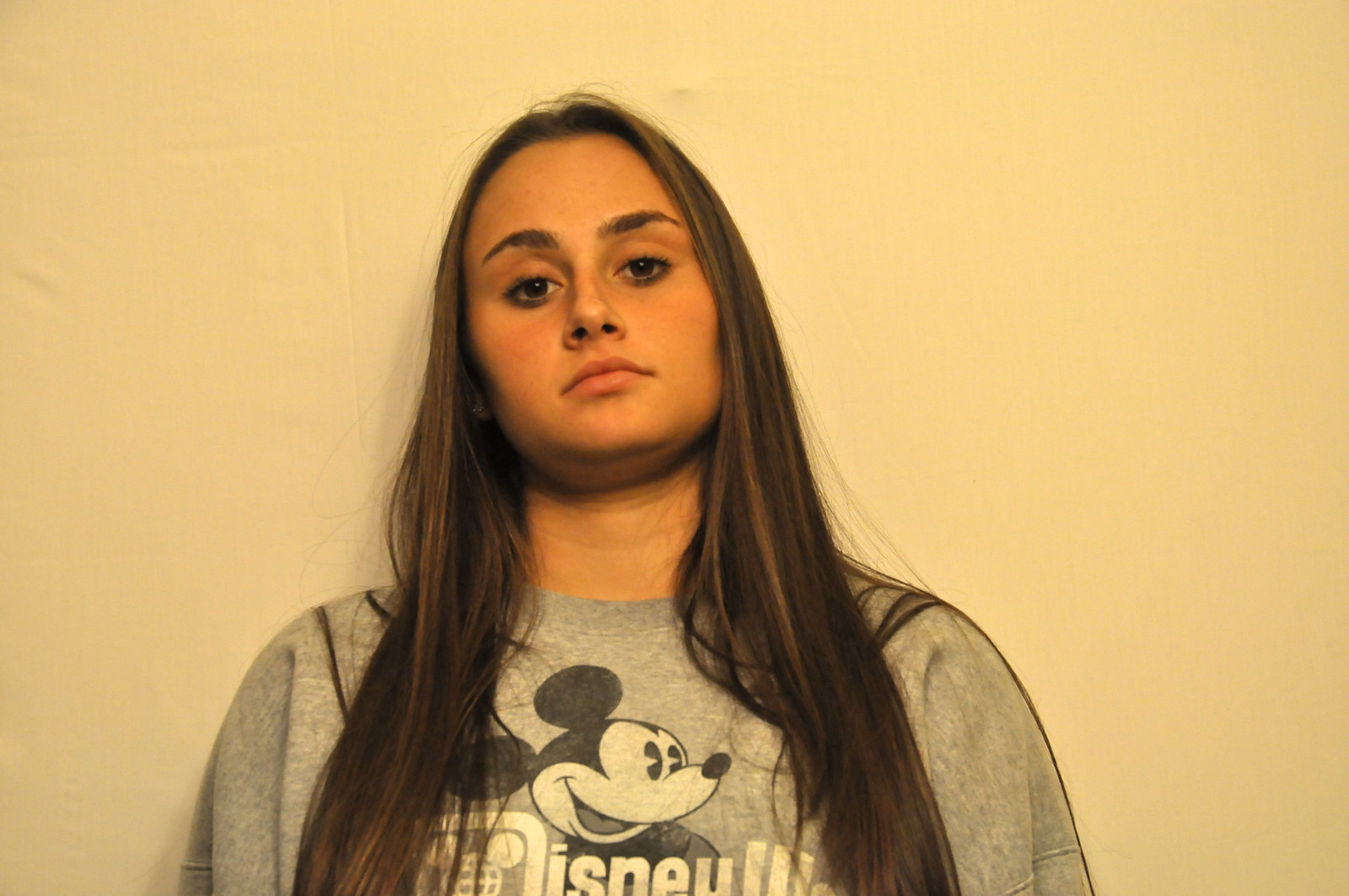In a warmly lit, indoor photographic setting with a slightly yellow and blue-tinted light on a beige, cream-colored background, a young woman in her late teens to early 20s stands against the wall. Her head tilts slightly from bottom right to top left, and her face shows a forlorn, somber expression. She has long, dark brown hair cascading past her shoulders down to her chest, framing her face with prominent dark eyes and thick eyebrows. She wears a gray t-shirt featuring a black and white graphic of Mickey Mouse facing to the right, with the iconic Disney text and logo printed underneath. The woman appears to have no makeup on, further emphasizing her natural, expressive features.